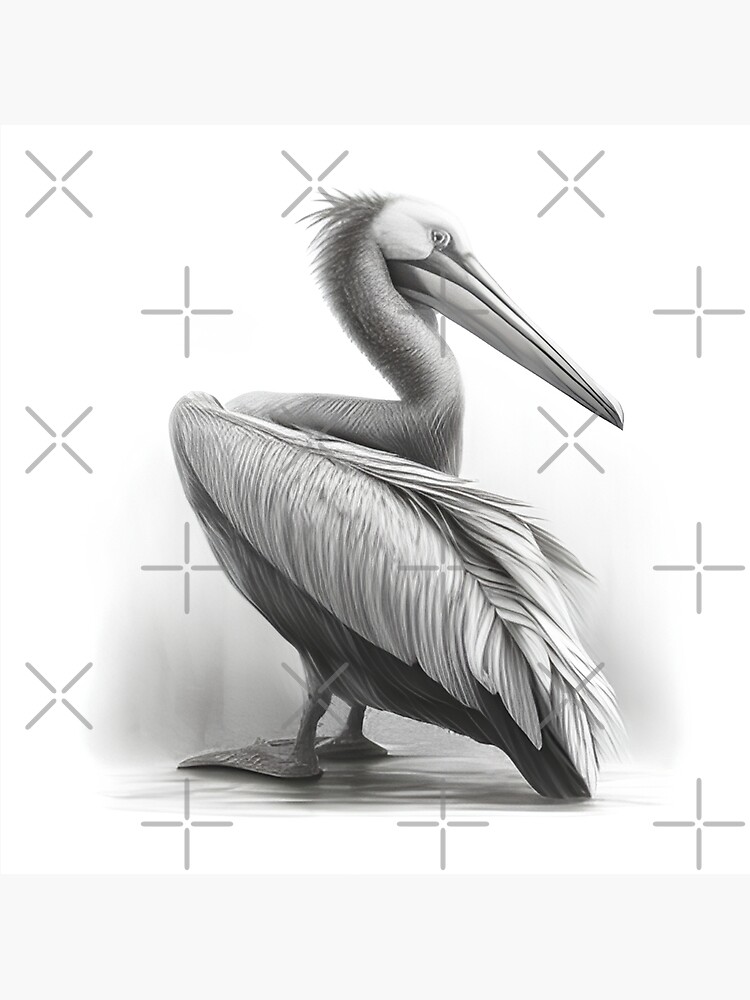This detailed black-and-white illustration depicts a pelican with its body facing away and to the left, while its head and long, curved neck turn to the right. The pelican's eye gazes directly at the viewer. The top of its head is white, transitioning to a darker shaded beak which spans nearly the width of its body. The neck, described as a backwards '2', shows a striking contrast with short hair that is white on the right and dark gray on the left. The bird's upper body feathers are predominantly white while the lower body is gray. Its feet, equipped with large triangular flippers, are pointed to the left. The background features a smoky gradient with a series of uniformly spread X's and plus symbols as a watermark, adding an additional layer of texture to the image.